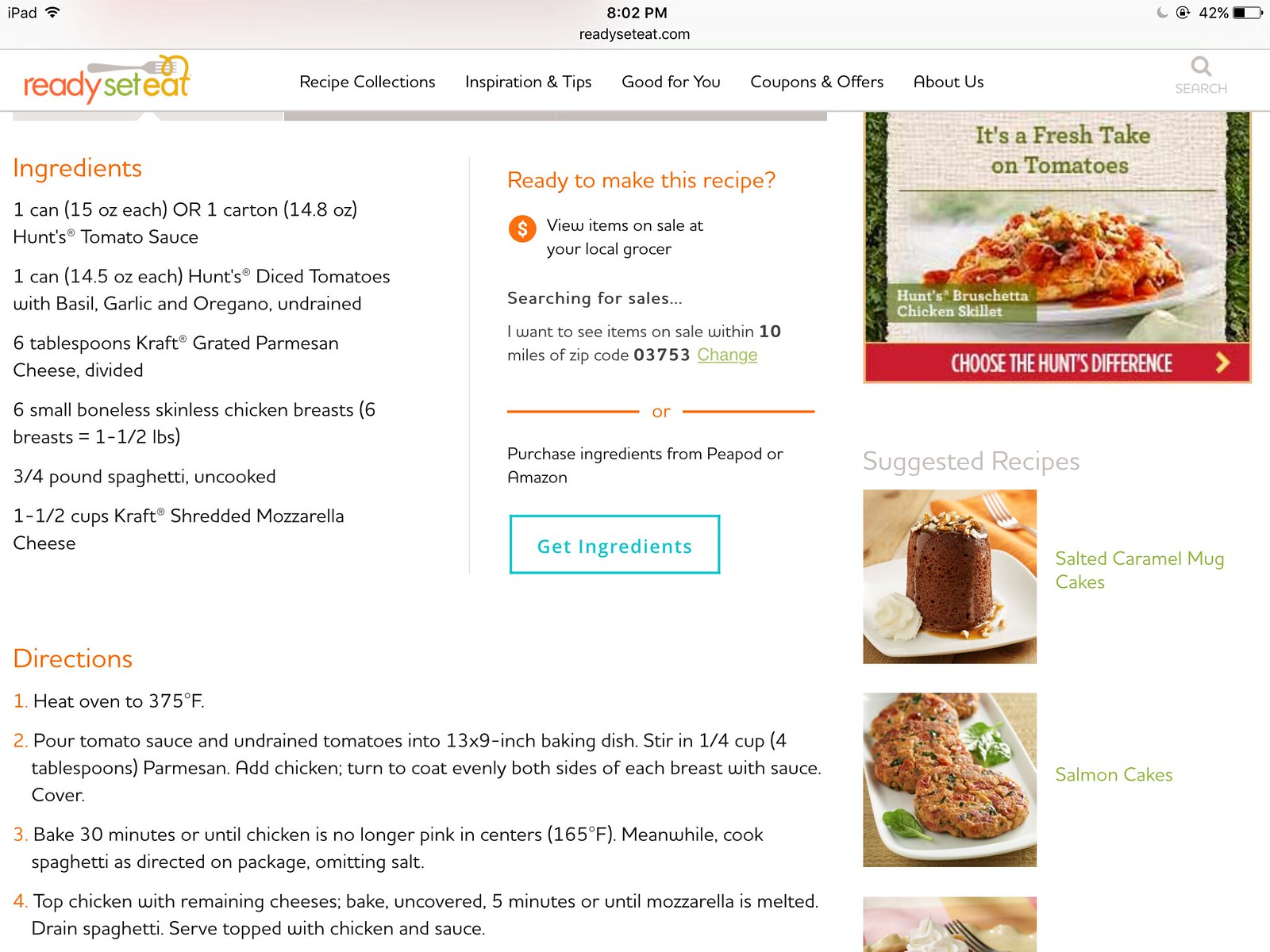This is a detailed screenshot of an iPad displaying a webpage at 8:02 p.m. with a battery level of 42%. The visited website is ReadySetEat.com, clearly indicated by the Ready, Set, Eat logo in the top left, which features a distinctive spaghetti noodle and fork design. The webpage includes a variety of menu items such as recipe collections, inspiration and tips, good for you, coupons and offers, about us, and a search button on the far right. The central content of the screen shows an unnamed recipe with a list of ingredients including tomato sauce, tomatoes, cheese, chicken, spaghetti, and mozzarella cheese. Directions for the recipe are provided below the ingredients. Additionally, the site features a column allowing users to shop for ingredients through Amazon. On the right side of the webpage, there is an advertisement promoting a fresh take on tomatoes with an option to try Huntz bruschetta chicken skillet, along with suggested recipes such as a salted caramel mug cake and a salmon cake.